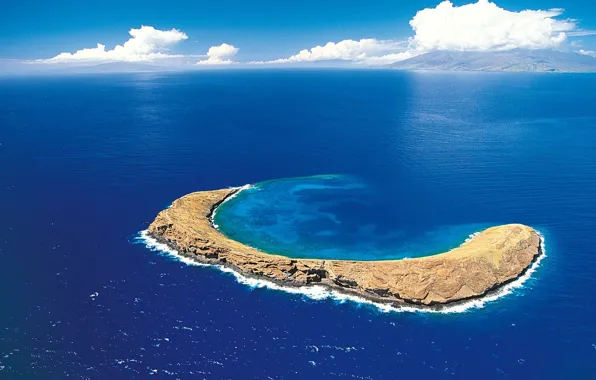The photograph captures a stunning and picturesque scene of a Pacific Ocean atoll. Dominating the foreground is a C-shaped rocky formation, enveloped by the warm, inviting expanse of the deep blue ocean. The image, crisp and vivid, showcases the surrounding turquoise waters, hinting at shallow areas and possibly coral reefs. The rocky edges are vividly detailed with white foam breaking against them. In the distance, partially obscured by some clouds on the horizon, stand majestic mountains, adding to the serene vista. The sky is a clear blue, dotted with a few white clouds, enhancing the tranquil and untouched nature of the scene. No people or additional objects are visible, emphasizing the pristine and isolated beauty of the atoll.